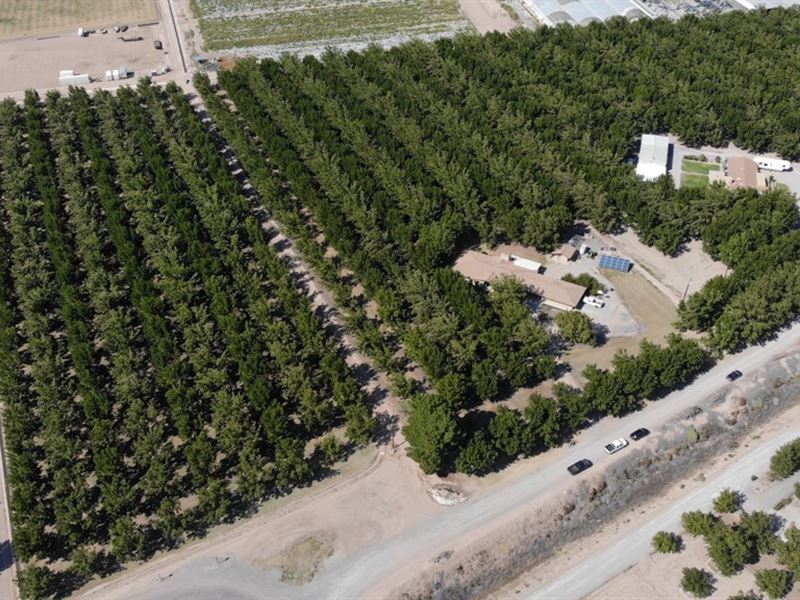This aerial photograph showcases a vast orchard with hundreds of neatly planted green trees stretching from left to right across the image. The trees are organized in evenly spaced rows, indicating deliberate cultivation rather than a natural forest. Nestled within the orchard are two large houses on the right-hand side, one accompanied by several vehicles, including a pickup truck, and another with a camper parked beside it. Additional buildings and clearing areas punctuate the sea of green, some featuring solar panels and white trucks. Roads weave through these clearings, with cars visible both within the orchard and along a prominent road in the bottom right, where four vehicles are lined up along the bushes across the street. The image also reveals further development beyond the orchard's borders, with more cars, streets, and greenhouses visible in the top right, blending the cultivated landscape with suburban elements.